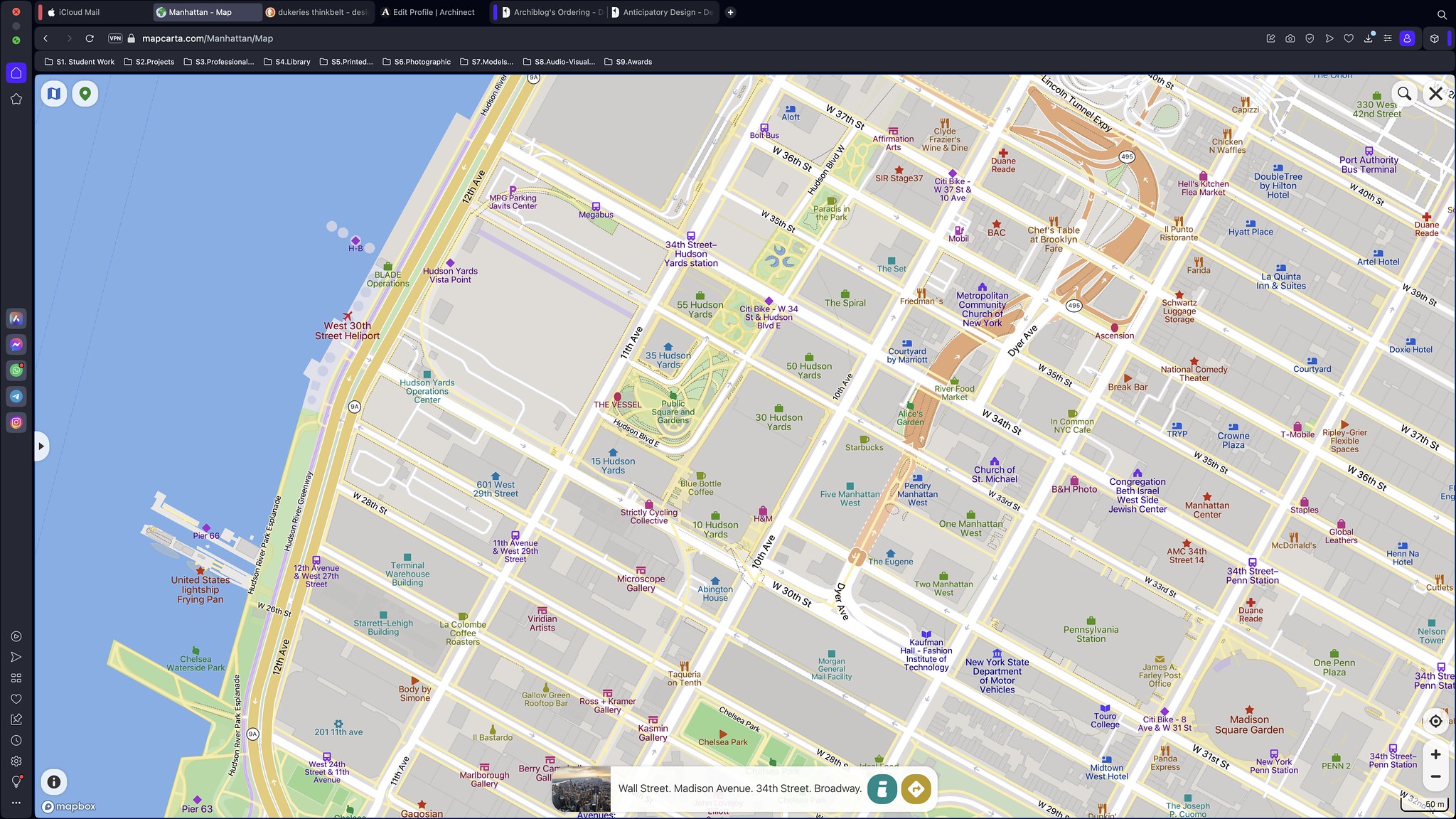A digital photograph captures the screen of a computer or laptop. On the left side of the screen, running from top to bottom, there's a black bar, complemented by another black bar running horizontally across the top. Both bars feature various icons. Starting from the upper left corner of the vertical bar and moving downward, there are blue, red, and green circles. Below these, there is a blue square containing a white symbol, followed by a generic house icon outline.

In the center of the screen, there are several colorful squares arranged next to each other. These squares are pink, blue, green, dark green, another blue, and another color that is unclear. At the bottom corner of this section, there are additional shapes including a circle, triangle, and a square resembling a heart. The rest of these shapes are blurry and indistinguishable.

At the top right of the screen, there are numerous open tabs for different websites, though their specific addresses are unclear. A large map application, possibly Google Maps, occupies a significant portion of the screen. 

On the left-hand side of the map, there is a vibrant blue area representing water, with white rectangles indicating piers. Adjacent to the water is a landmass with a prominent dual-lane yellow road, likely a highway, surrounded by numerous streets running in both north-south and east-west directions. A central road stands out in orange, suggesting another major thoroughfare. Various markings in blue and green are scattered throughout the map.

Near the bottom, there's a white rectangle with black text that is illegible, accompanied by blue and green circles. In the bottom right corner, there's a rectangle containing a plus and minus sign, presumably for zooming in and out of the map.